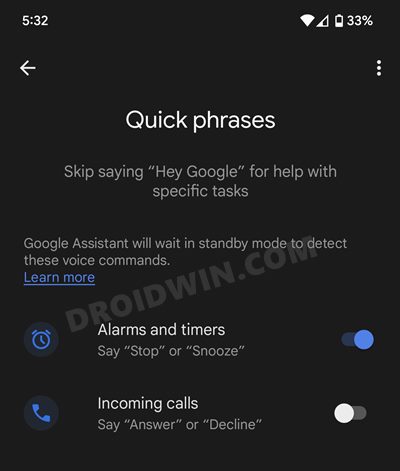The image displays a primarily black background with a rectangular section at the top containing various status indicators and text. In the top right corner, white icons show the time as 5:32, a Wi-Fi signal, a cellular signal, a battery icon, and the battery percentage at 33%. Below this header, on the left side, there is a left arrow, and on the right side, there are three small vertical dots arranged in a column.

Centered below this header section, the text "Quick Phrases" is displayed with a capital "Q". A lighter text underneath reads: "Skip saying 'Hey Google' for help with specific tasks." Following this is a paragraph explaining, "Google Assistant will wait in standby mode to detect these voice commands."

Further down, a clickable blue underlined text reads "Learn More."

Below this, there is a section with a blue circular icon featuring an alarm clock and labeled "Alarms and timers." It instructs the user to say "stop" or "snooze" (with both commands in quotations) and indicates that this feature is enabled by showing a filled blue circle on the right side.

Next, another section features a blue circular icon with a phone, labeled "Incoming calls." It advises to say "answer" or "decline" (with both commands in quotations) and shows that this feature is turned off, as indicated by an unfilled circle on the right side.